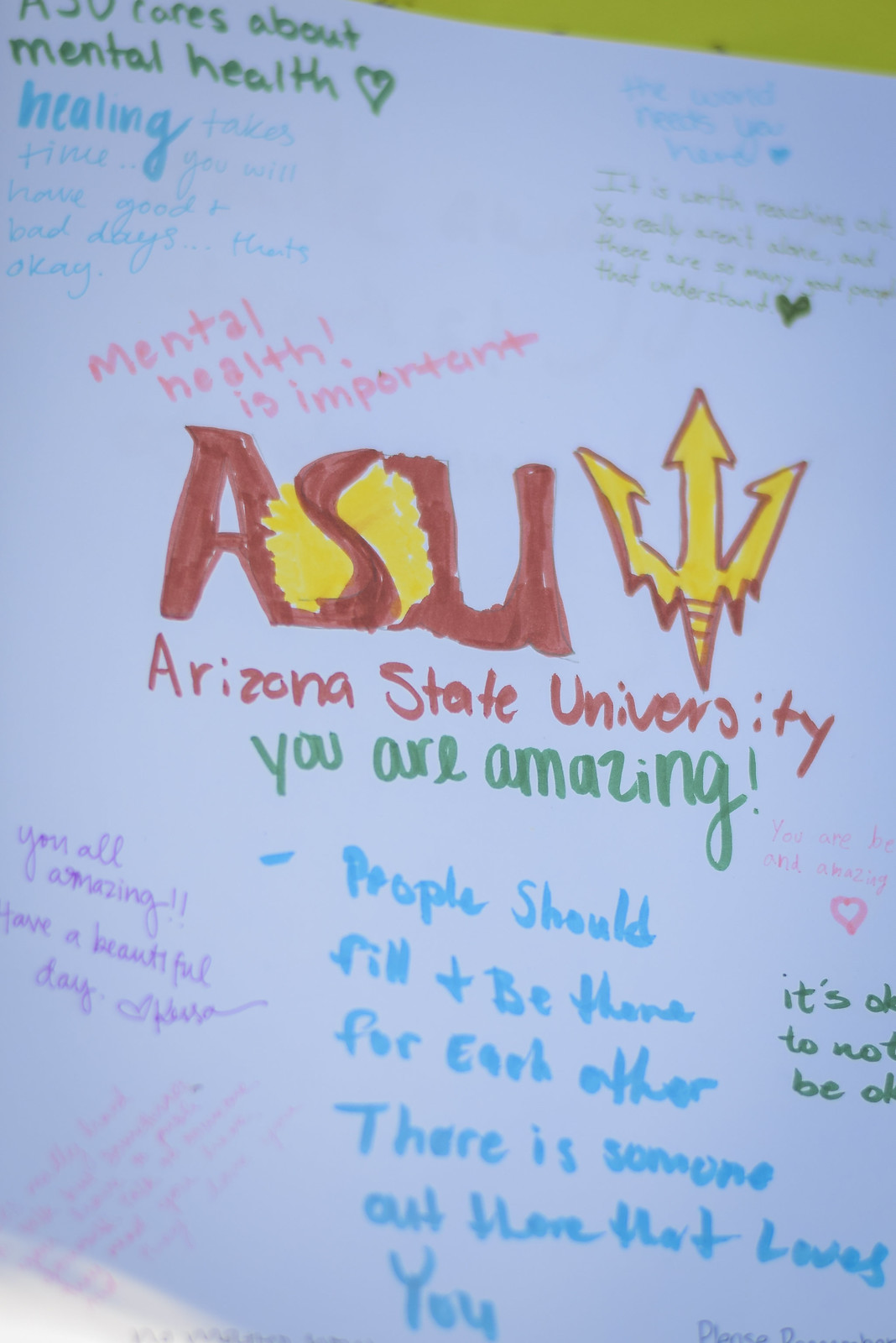The image is a detailed, colorful poster dedicated to mental health encouragement at Arizona State University (ASU). At the center, the iconic ASU logo is prominently displayed in red, featuring the letters ASU with a yellow sun behind the 'S' and a triangle in yellow and red beside it. Just below the logo, "Arizona State University" is written in red, followed by the uplifting message, "You are amazing!" in green. 

Above the ASU logo, a message in pink reads, "mental health! is important." Scattered across the poster are various handwritten notes in different colors. One of the legible notes, written in blue beneath "You are amazing!" states, "people should feel and be there for each other. There is someone out there that loves you." Another note emphasizes, "healing takes time, you will have good days and bad days, that's okay." The background appears to be filled with additional encouraging messages, making this poster a heartfelt testament to community support and mental health awareness at ASU.